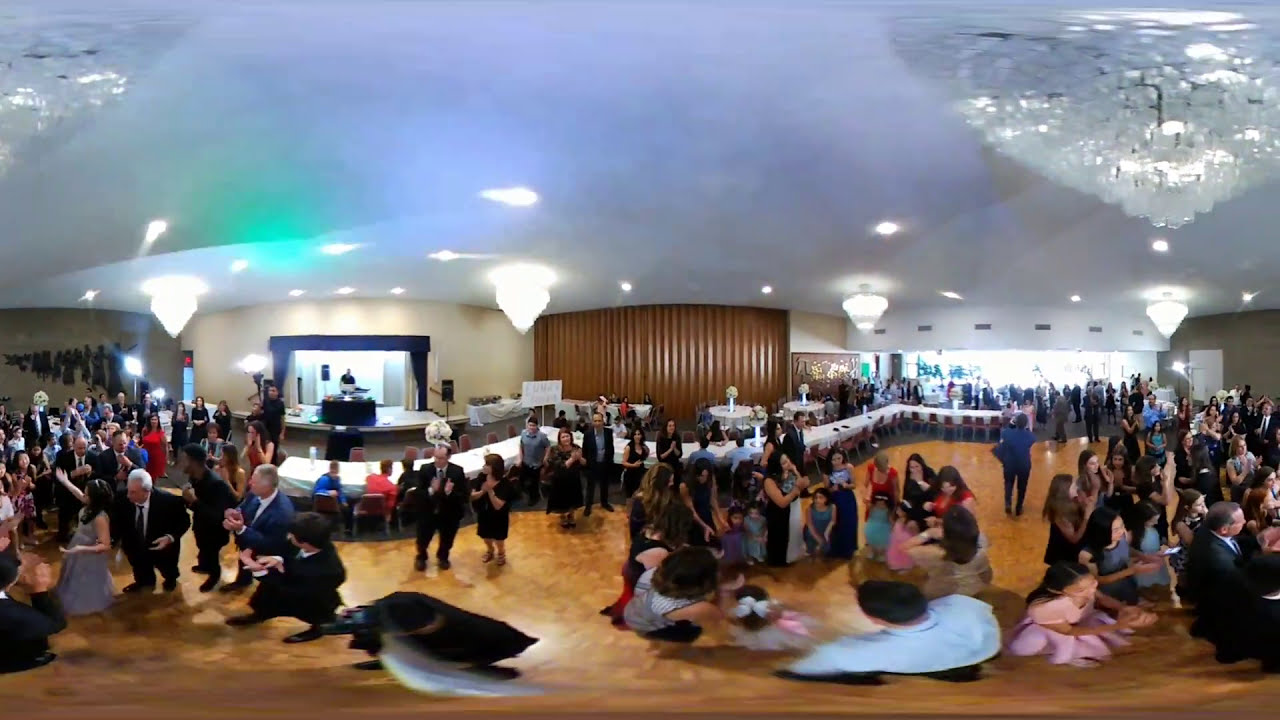This indoor photograph captures what appears to be a formal event, possibly a wedding or a large gathering, situated in a grand auditorium or similar venue. The spacious room features a polished brown floor, alongside a white ceiling adorned with multiple chandeliers. Notably, there are two large crystal chandeliers in the upper corners of the image and four smaller, bright white chandeliers lined up mid-frame from left to right.

The ambiance is elegant, with men dressed in suits and ties and women wearing long dresses. A long table covered with a white tablecloth is prominently placed, surrounded by chairs, suggesting either a dining arrangement or a check-in area. Some people are seated at the table, while a majority are standing, with many appearing to be clapping, indicating an ongoing celebration or a notable moment in the event.

In the background, a brown curtain adds a touch of formality to the setting. At the lower right corner, a group of people faces towards the right, whereas others are positioned as if captured mid-conversation or interaction. The image appears to be a composite, creating minor distortions with tables and walls displaying bends and curves. Overall, the scene is filled with well-dressed attendees, immersed in an atmosphere of elegance and celebration.